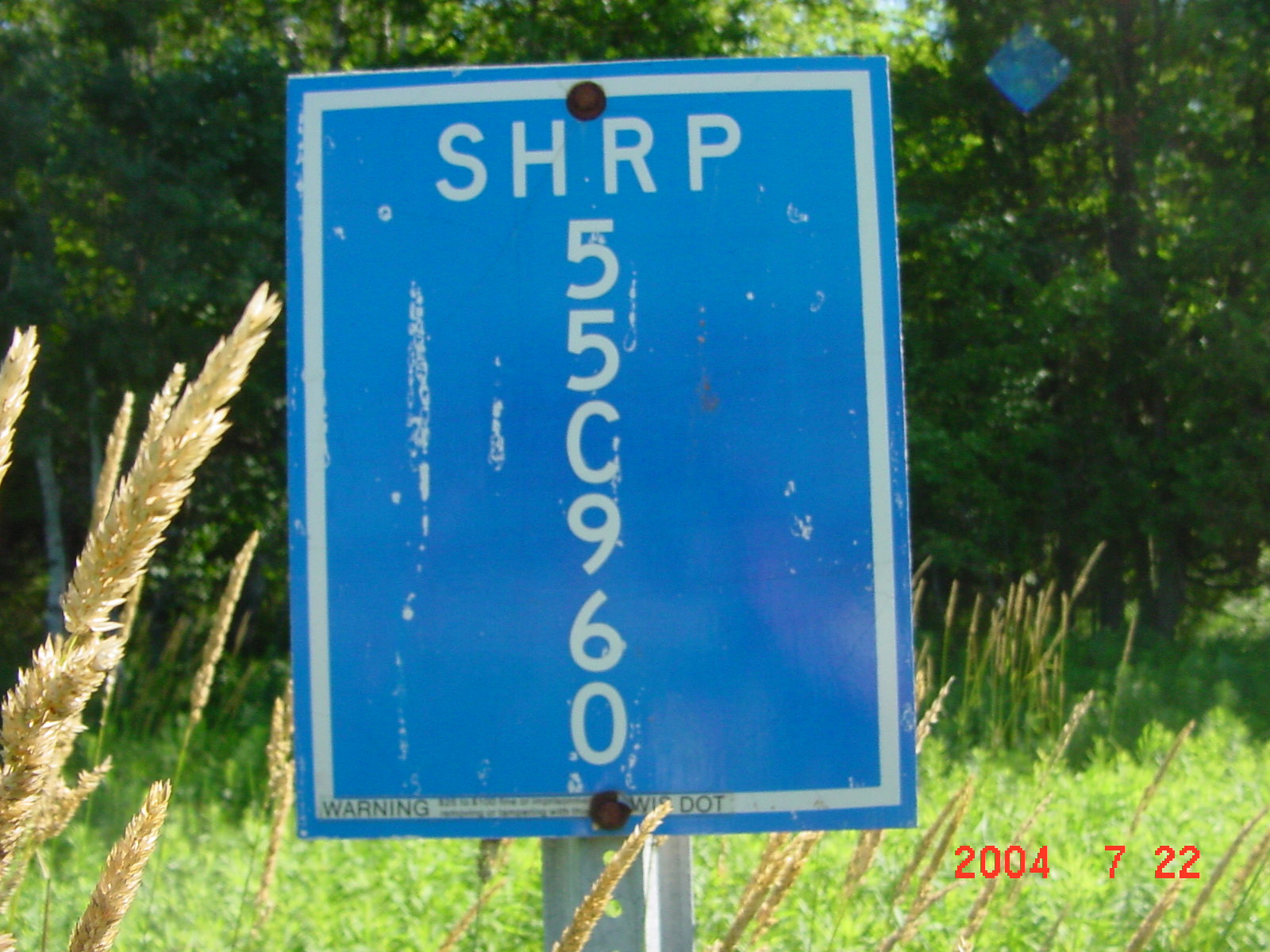A vibrant blue rectangular roadside sign stands prominently amidst a grassy verge, illuminated by bright sunlight. The sign features a mix of numbers and letters in bold white font, with a clear, distinct border framing its edges. Mounted on sturdy metal posts, the sign is secured with two large fixing nuts. Below, text including "D.O.T." is partially visible, though its full message is obscured. The scene is set against a backdrop of dark, shadowy trees that contrast with the sunlit grass in the foreground, highlighting the sign's importance and the surroundings' natural beauty.